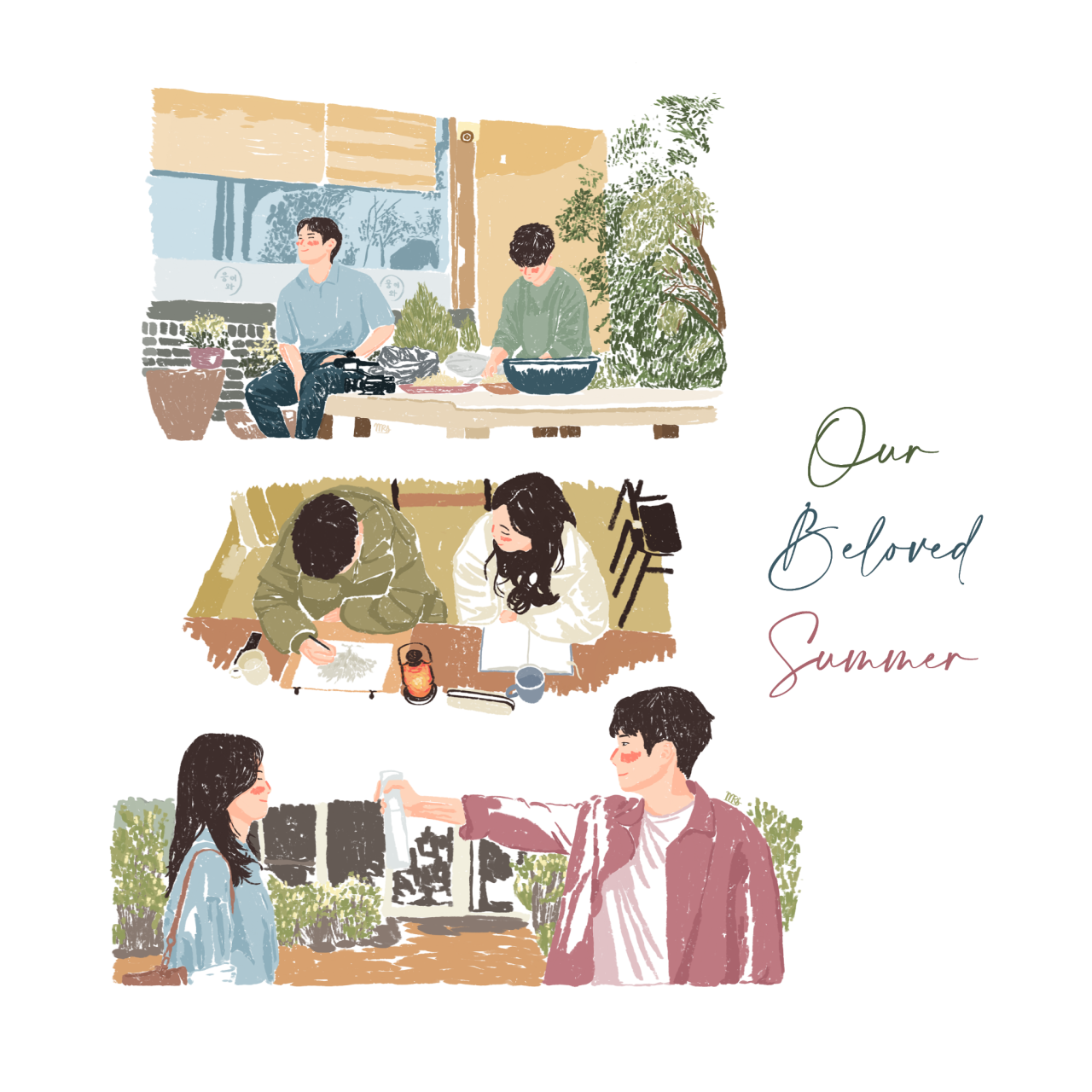The drawing features a triptych arrangement with three distinct scenes, each encapsulated within a rough, non-linear border that lacks a straight edge. 

**Top Image:** This scene depicts two people sitting at a picnic table, likely situated in front of a school or another type of building. The figures are engaged in a conversation or activity, providing a sense of connection and casual interaction.

**Middle Image:** The viewpoint shifts to an aerial perspective, capturing two individuals seated at a desk or bench, with books sprawled out in front of them. This bird's-eye view offers a unique insight into the shared space and activity of the subjects, suggesting a scholastic or collaborative environment.

**Bottom Image:** The final scene shows two people facing each other, viewed from the side. The individual on the right has his hand extended, possibly in a gesture of greeting or offering something. This interaction adds a dynamic element to the composition, reinforcing themes of communication and relationship.

Throughout the drawing, the text "Our Beloved Summer" is inscribed, adding a nostalgic or sentimental layer to the overall theme.